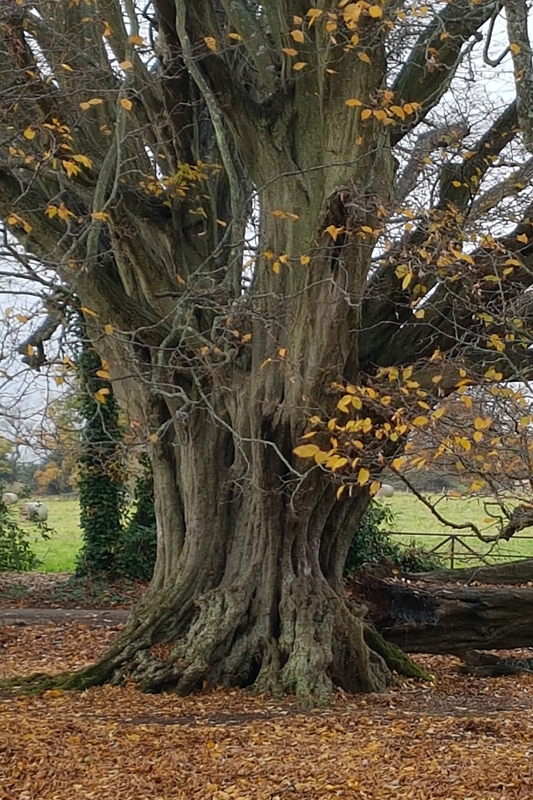In this captivating autumnal photograph, we see a thick, mature tree standing proudly in a serene setting. The scene is bathed in the warm hues of fall, with golden-yellow leaves clinging to the outstretched branches, while the majority have carpeted the ground below, now browned with age. The tree's robust trunk showcases numerous crevices and separations, almost as if ten trees were melded together, emphasizing the intricate beauty and resilience of nature. Some of its roots venture above the ground, snaking away from the base and adding texture to the composition. In the background, a lush grass lawn extends into the distance, interrupted by a glimpse of a fence on the lower right and a few rounded bales of hay resting in the field beyond, hinting at a pastoral landscape.